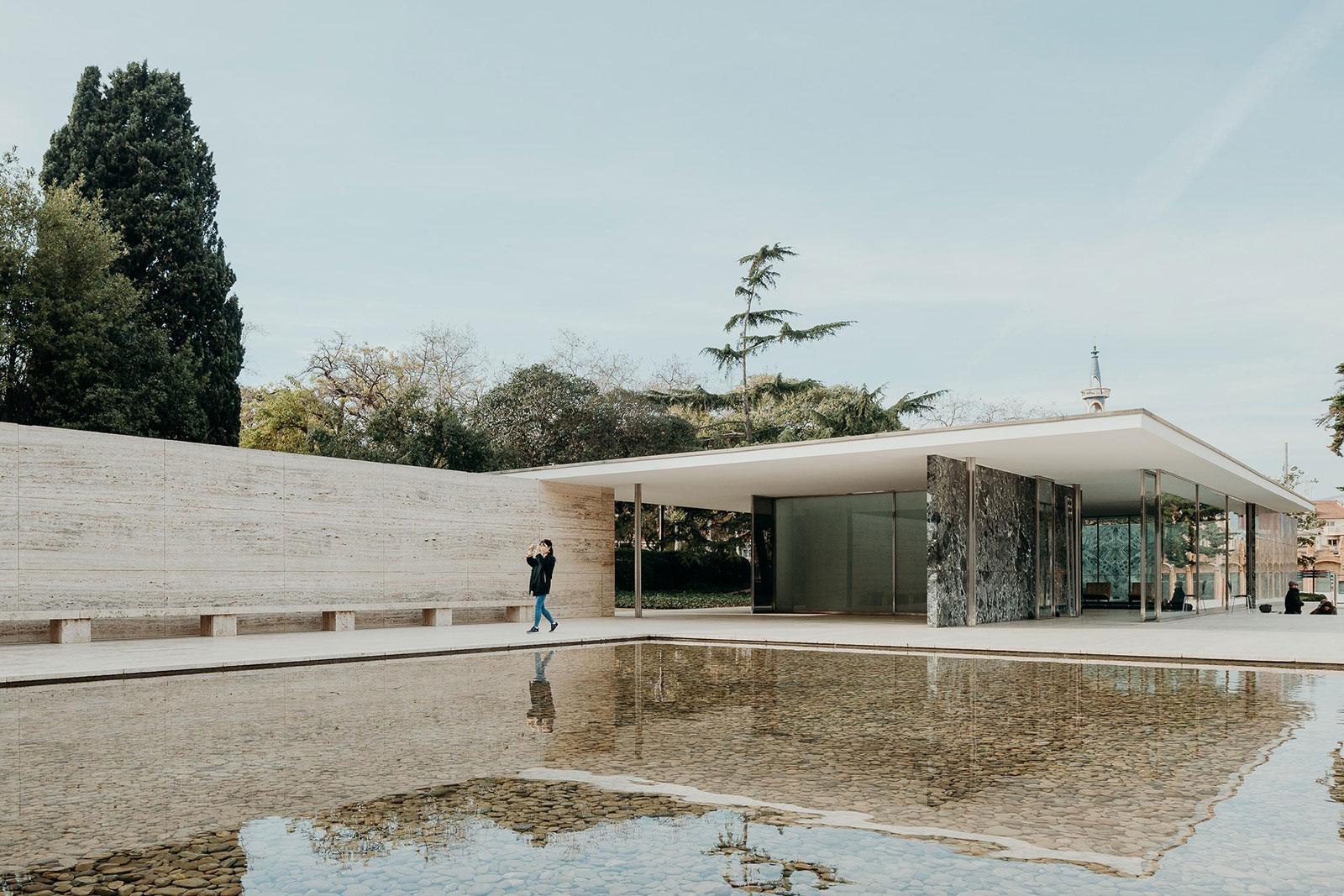This outdoor photo features a strikingly modern structure, characterized by simple, minimalist architecture reminiscent of Mies van der Rohe's style. Dominating the image is a long, sleek, concrete wall that extends beneath an awning, creating a partially covered open space that appears ideal for placing a picnic table or for communal gatherings. The structure itself is predominantly made of glass, with large windows that emphasize its modernist aesthetic. Adjacent to the glass-walled building is a serene reflecting pool filled with stones, which mirror the building and create a sense of tranquility in the composition.

A walkway runs alongside the wall, bordered by this reflective body of water. On this path, a person in blue pants and a dark jacket strolls by, though they are barely discernible as they are far in the background. The scene is set under a bluish-gray sky, adding a cool tone that complements the clean, modern lines of the architecture. The background is dotted with evergreen trees, suggesting a season of early spring or early fall. There is a suggestion that the long wall might be part of a tribute or memorial, given the presence of a person possibly taking a photograph of it. The building, with its flat roof and extensive use of glass, stands as a testament to modern design, possibly a pavilion or a symbolic piece from a World's Fair.